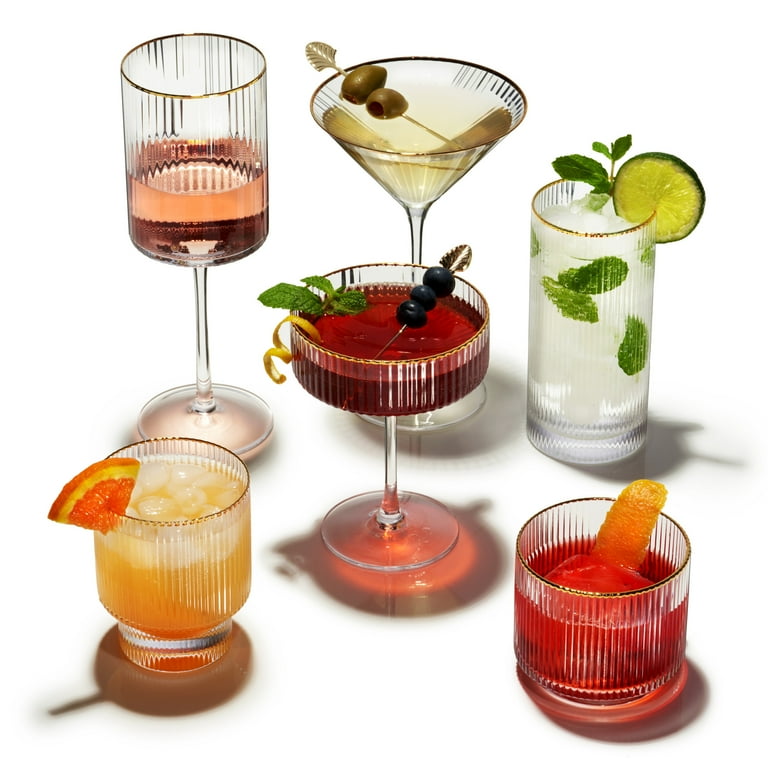The image showcases six various glass beverages, each contained within glasses of differing shapes and sizes but unified by a vertical ridged design and a gold rim around the top, suggesting they are from the same manufacturer. The top left glass is short and cylindrical, containing a pink, rose-colored liquid that resembles wine. The glass next to it is a wide, round-topped martini glass with a long stem, garnished with a toothpick of two olives. The central glass holds a dark red cocktail, possibly cranberry juice, with blueberries floating in it. To the right is a mint julep-like beverage with a whitish liquid, mint leaves, and lime. The front left glass holds an orange-colored drink, likely orange juice, adorned with an orange slice and filled with ice. Lastly, the glass on the front right contains a red liquid, perhaps cranberry juice, with ice and an orange peel garnish.